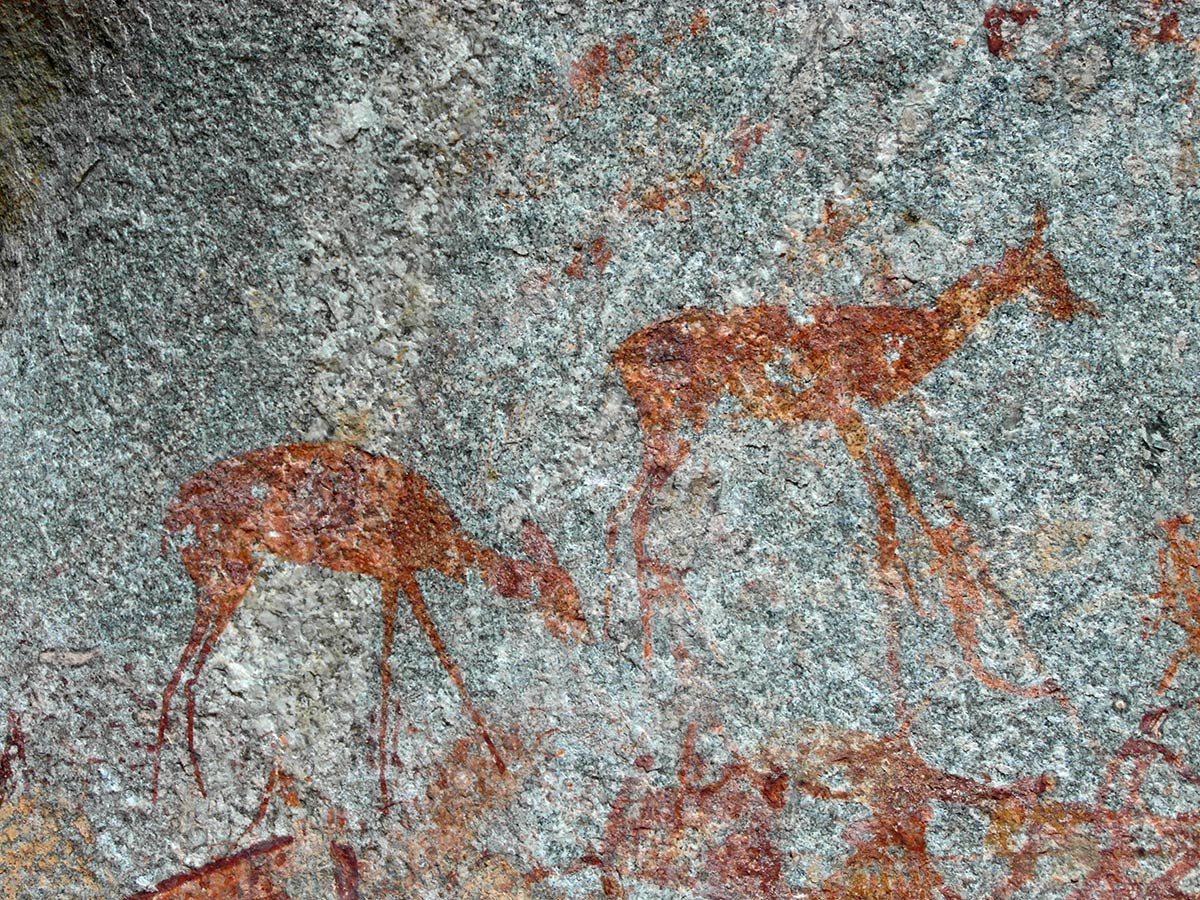This image captures an ancient drawing on a cave wall from a previous century, resembling antique cave art. The rock surface is a mix of silver, white, light grey, and dark grey hues, providing a contrasting backdrop to the artwork. The detailed drawing, rendered in dark red, brownish, or rusty orange tones, depicts two animals that resemble deer or antelopes with long legs and ears, and notably lacking tails. The animal on the left is depicted with its head bowed, as if grazing, while the one on the right stands more upright, looking off to the side. Additional rudimentary markings or scribbles are visible at the bottom of the image, further emphasizing the ancient and historical nature of the scene.